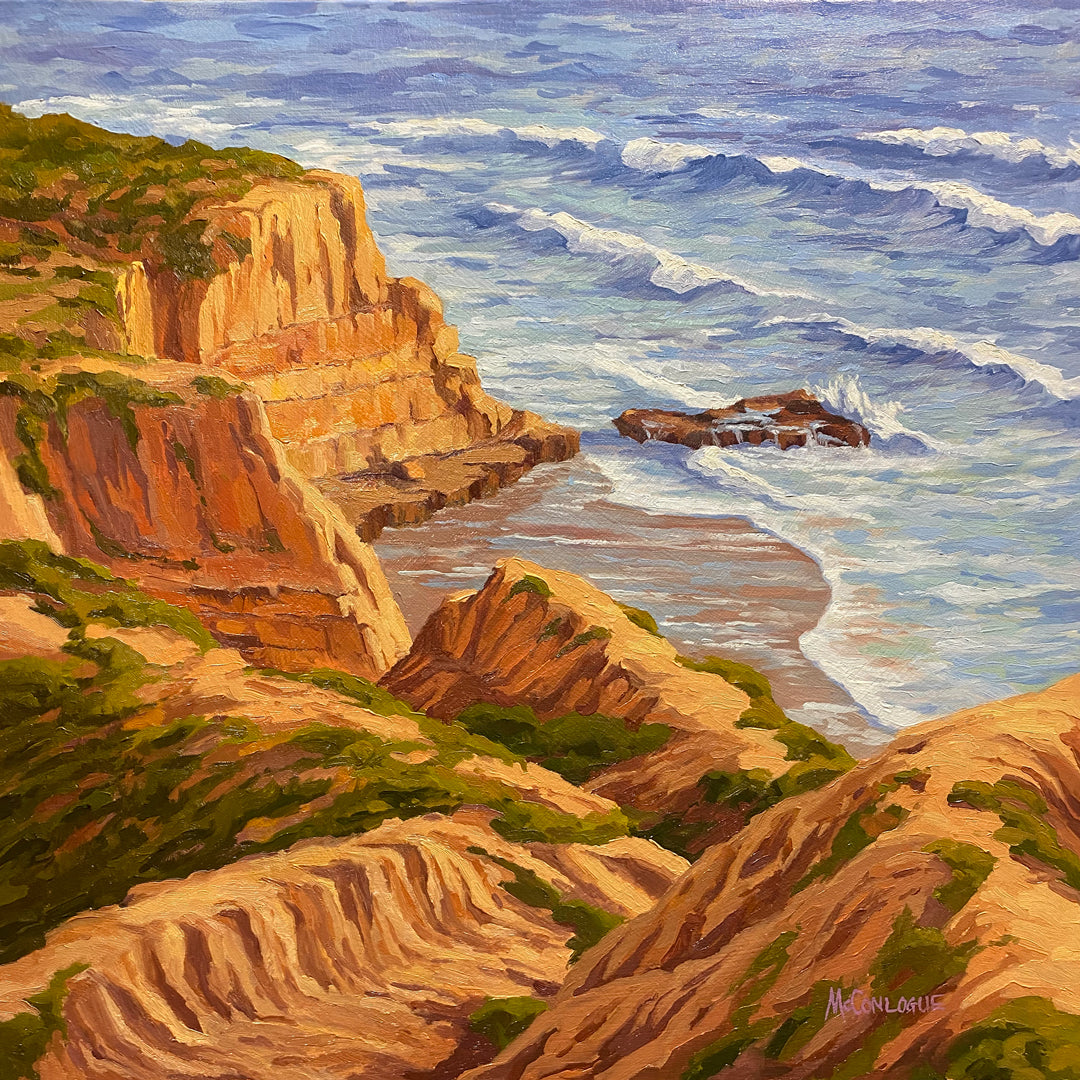This vertical, rectangular impressionistic oil painting depicts a dramatic coastal landscape reminiscent of Cezanne's use of color and form. The foreground features sprawling golden-brown cliffs that dominate the bottom and the left side of the image. These cliffs, imbued with hues of orange, yellow, and brown, stretch from the bottom almost to the top, forming a rugged barrier. Nestled within these cliffs, a small, inviting beach appears, its sands bordering a light blue, choppy sea. The ocean, marked by white, foamy waves crashing onto the shore, fills the top and right portion of the canvas. Notably, in the mid-right section of the scene, a lone rock juts out into the water, enduring the relentless breaking waves with colors matching the adjacent cliffs.

Interspersed along the cliff tops are splotches of green, representing stylized bushes and grass, adding an element of vibrancy. The sea features soft, yet deliberate white brushstrokes indicating the movement of waves as they wash onto the sand and up against the rock face. Visible on the lower portion of the painting, there is an indistinct signature, likely "Mick Conlogue," rendered in light pink, adding an authentic touch to this piece. Despite its somewhat amateurish and cartoonish elements, this painting effectively captures the essence of a seaside cliff with a blend of stylized and realistic components.